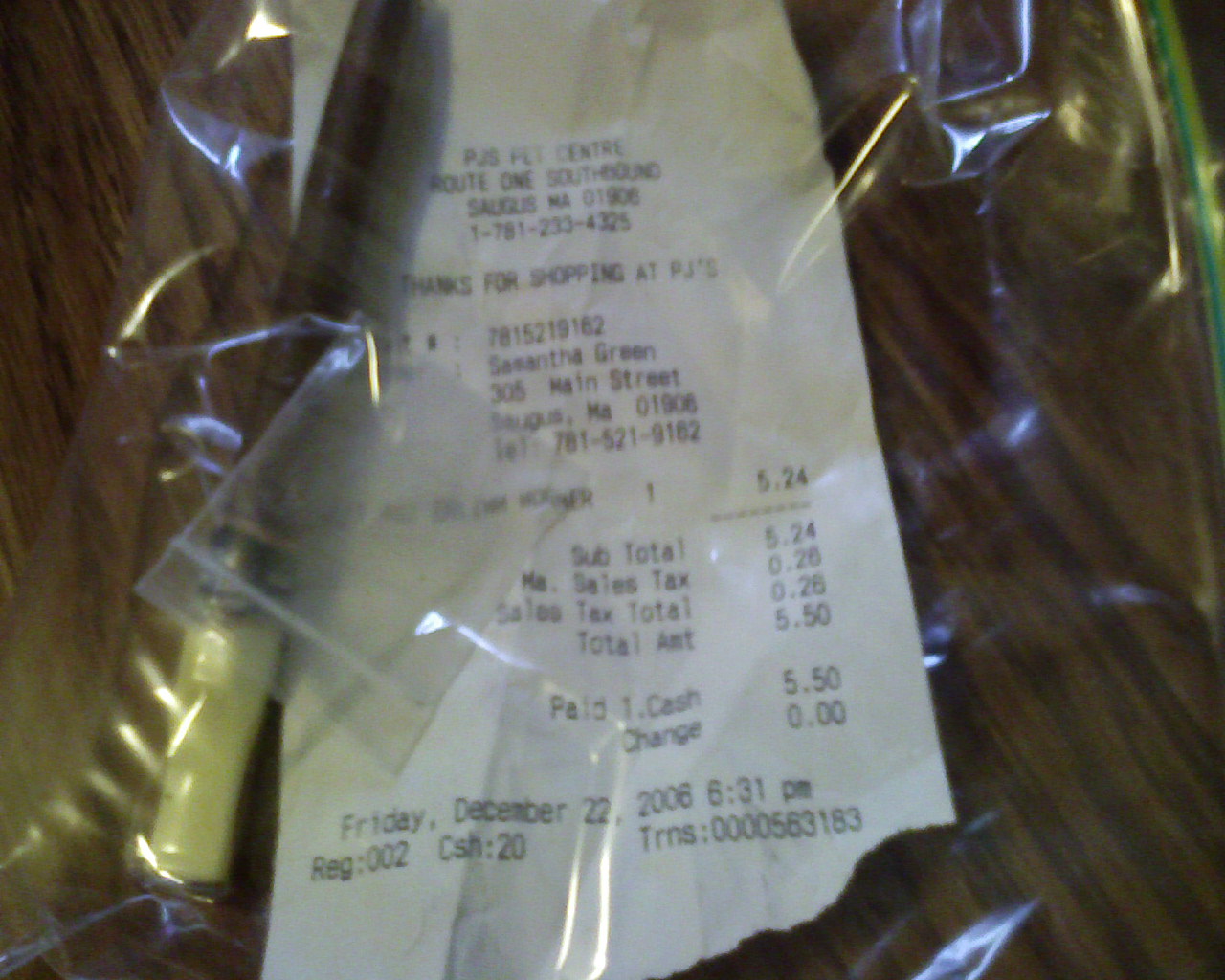This horizontally-oriented, rectangular image captures a number of items arranged on a brown wood-stained tabletop. Dominating the center, running vertically from top to bottom, is a white receipt with black print. The receipt displays the following details: "Pet Center, Route 1, Southbound, Saugus, Massachusetts, 01906, Phone Number 1781-233-4325", and concludes with the message "Thanks for Shopping at PJ's". Notably, the amount paid, $5.50 in cash, is highlighted at the bottom right corner of the receipt.

Overlaying the top of the receipt is a transparent plastic bag, partially obscuring the details. To the left of the receipt lies an object resembling a long knife, featuring a dark blade and an ivory-colored handle. This intricate arrangement of items resting on the brown wood-stained surface creates a compelling tableau that captures the viewer's attention.